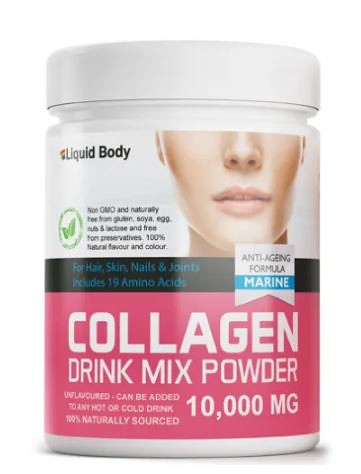The image portrays a plastic bottle featuring a screw-off white lid, predominantly white and pink in color. The bottle prominently displays the lower half of a woman's pristine face, showcasing her nose, lips, and upper neck. Above the image, in black letters, the brand name "Liquid Body" is inscribed. The bottle is labeled as a "Collagen Drink Mix Powder," providing 10,000 milligrams of collagen. Emphasizing its benefits for "hair, skin, nails, and joints," the product boasts an anti-aging formula and includes 19 amino acids. The background beneath the main text is pink with large white lettering, while smaller text highlights that the powder is unflavored and can be added to any hot or cold drink. Remarkably, the formulation is 100% naturally sourced, non-GMO, and naturally free from gluten, soy, eggs, nuts, lactose, and preservatives. An additional black ring around the jar includes further details about its natural flavor and color.